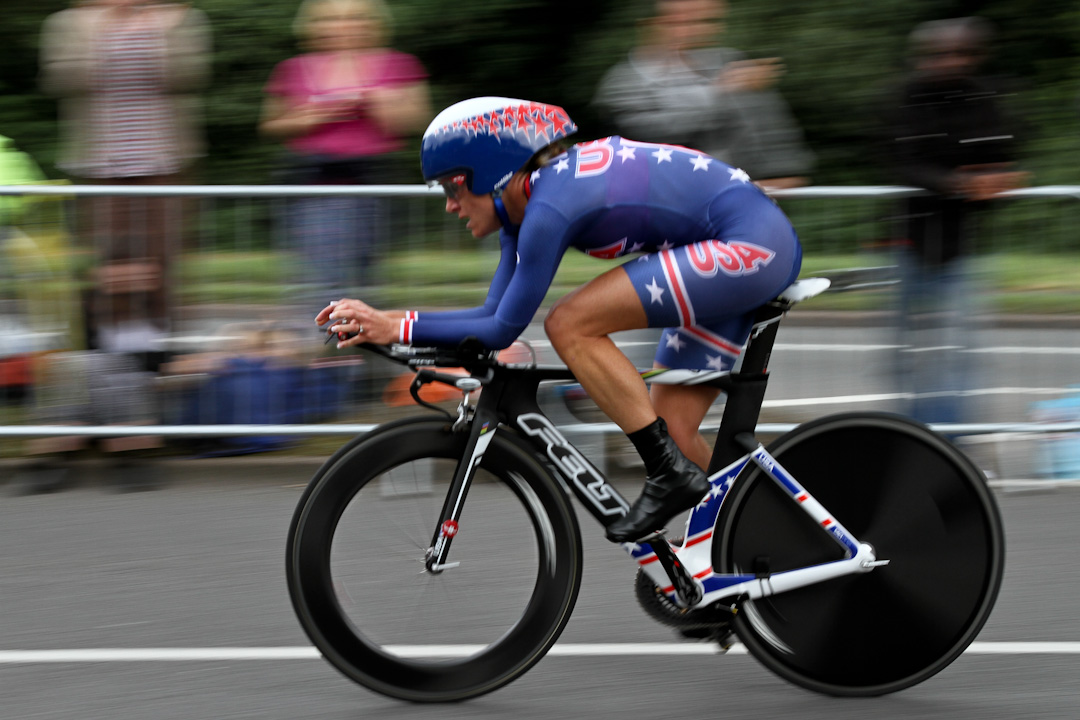This photograph captures a dynamic moment of professional bicyclist Kristen Armstrong speeding past a backdrop of blurred spectators and metal fencing. The focus is sharply on Armstrong, who is seen in a streamlined posture, hunching forward with forearms and hands gripping the handlebars. She is donning an aerodynamically shaped helmet and a tight blue spandex bodysuit emblazoned with the USA insignia, featuring red stripes and white stars. A wedding ring glints on her finger, adding a personal touch to her racing gear. Armstrong's bike, adorned with the logo "F-E-L-T" and highlighted by red, white, and blue striping, emphasizes the patriotic theme. The back wheel is solid black, contrasting with the semi-transparent front wheel, and both wheels have extremely thin treads, indicative of a high-performance racing bicycle. The combination of the focused cyclist and the motion-blurred background underscores the high speed and competitive nature of the scene.